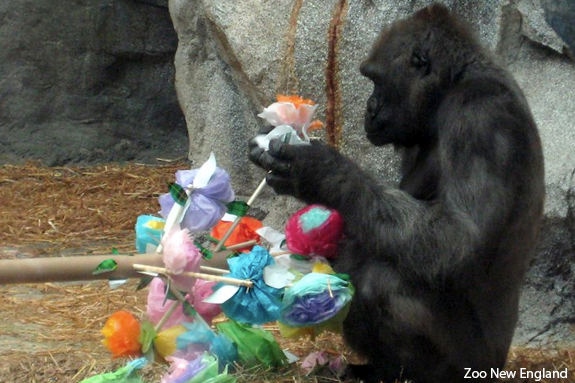The image captures a dark-furred gorilla, seated with knees in front, at Zoo New England. The gorilla is holding a white and orange paper flower in its hands, a part of a vibrant bouquet crafted from arts and crafts materials showcasing hues of purple, pink, blue, green, yellow, and orange. The animal is positioned against a backdrop of light to dark gray boulders, with a sparse layer of hay and mulch covering the ground. Additionally, a piece of bamboo is visible on the ground near the gorilla. The setting appears to be outside the entrance to a cave, suggested by an opening between the rocks. The text "Zoo New England" is inscribed in white in the bottom right corner of the image. There are no other people, animals, or identifiable objects in the frame.